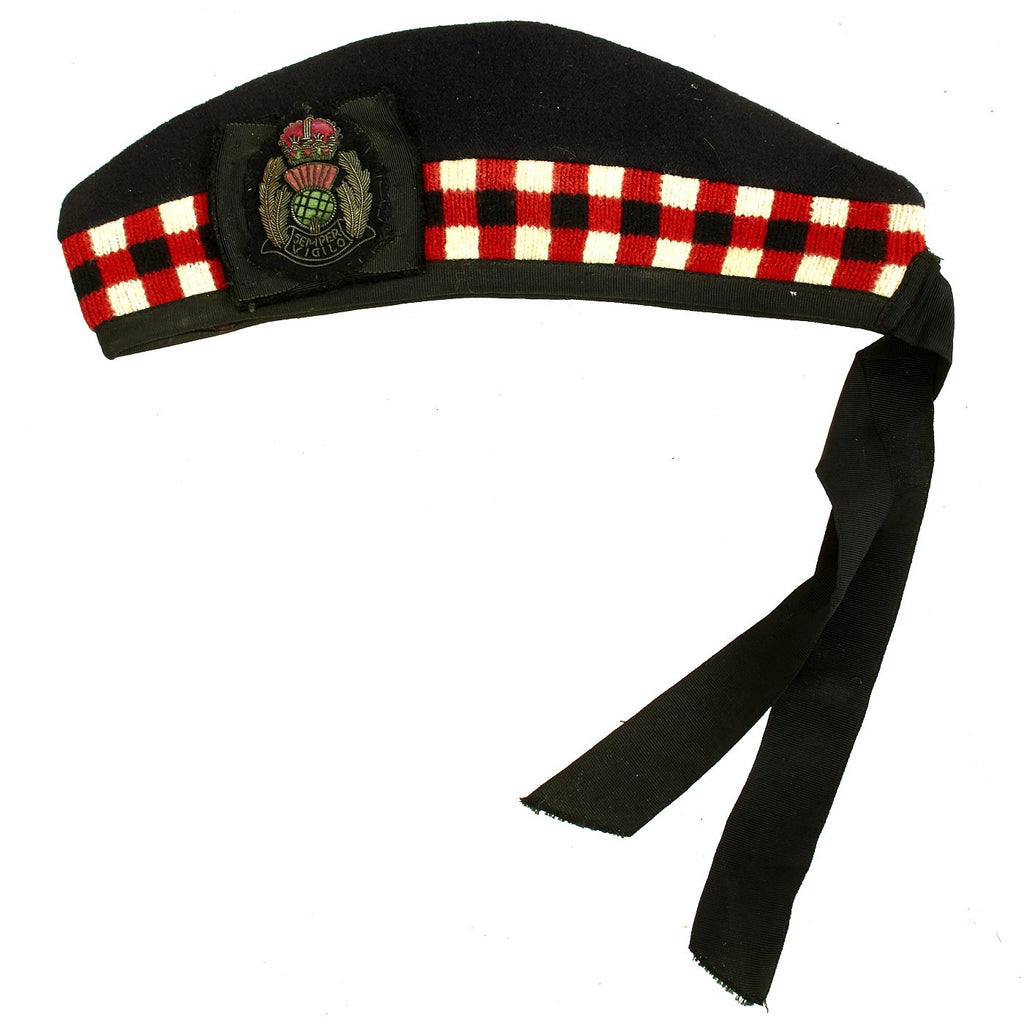The image depicts a flat, round, primarily black fabric hat that appears to be knit or handmade. The rim of the hat is black, which transitions into a distinctive checkered design composed of red, white, and black squares resembling a plaid pattern. This pattern forms a band around the middle of the hat, which is flat on top. At the front center of the hat is an intricate emblem featuring a crown at the top, with a green circular shape in the middle, possibly adorned with ferns or feathers, and a small banner with the words "Semper Viglio." Additionally, there are two long black strings hanging down from the back of the hat, and a black satin bow directly beneath the emblem. The details suggest that the hat may have some ceremonial or decorative significance.